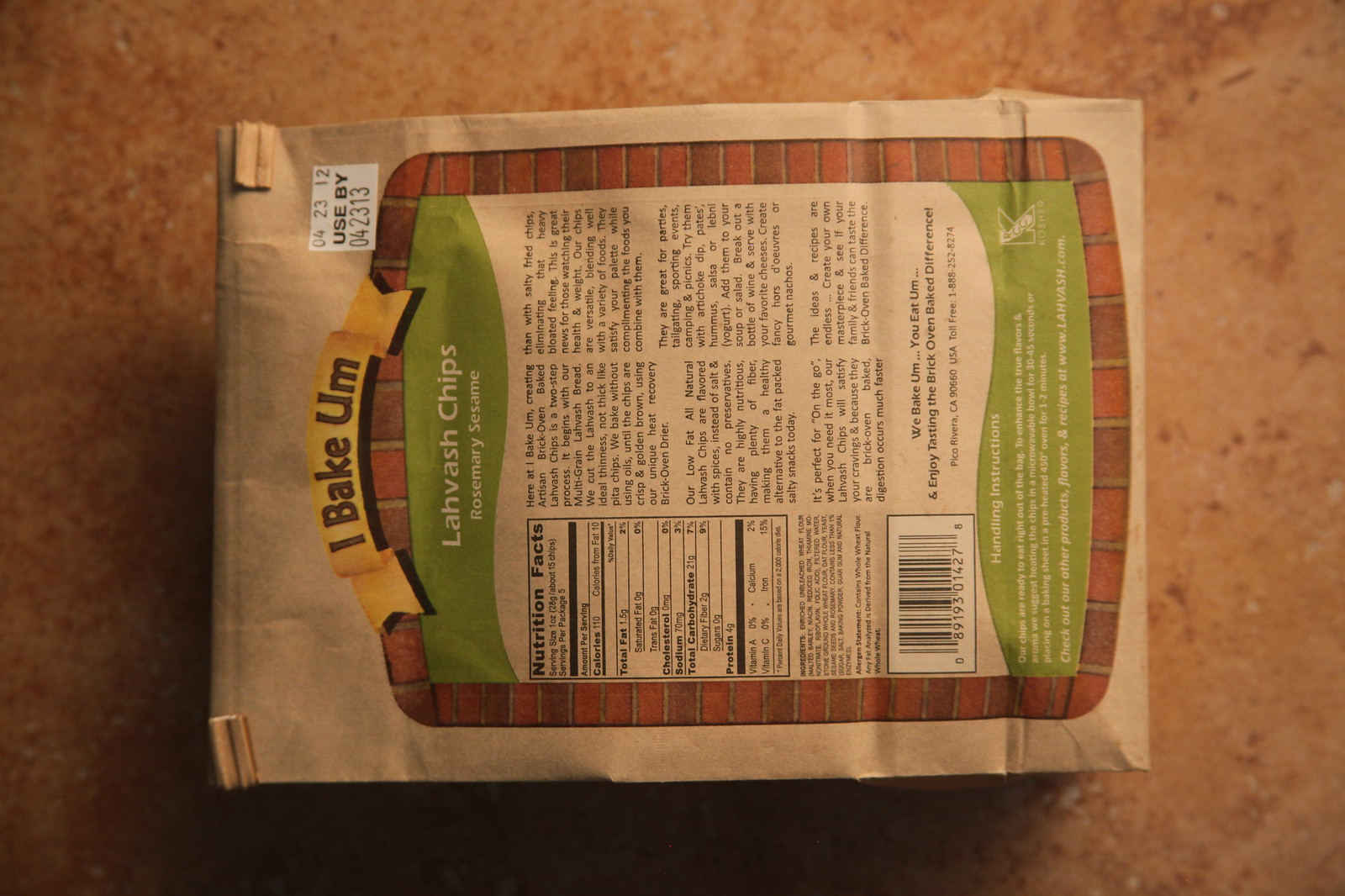This image is a horizontally displayed photograph of a bag of lavash chips on a dark brown, speckled countertop. The bag is supposed to be viewed vertically and prominently features a label at the top with the phrase "I bake them" set against a yellow background. A white sticker in the top right corner displays a use-by date of April 23, 2013. The bag is primarily tan with a green background section and white writing, accentuated by a brick pattern around the perimeter. These artisan rosemary and sesame-flavored chips, produced in Pico Rivera, California, are described in detail on the packaging. The description explains that the chips are made from multigrain lavash bread, cut thin, and baked in a unique heat recovery brick oven dryer until they are crisp and golden brown, without using oils. Additionally, there is a nutritional label and various other pieces of informational text throughout the packaging, reinforcing the artisanal nature of the product.